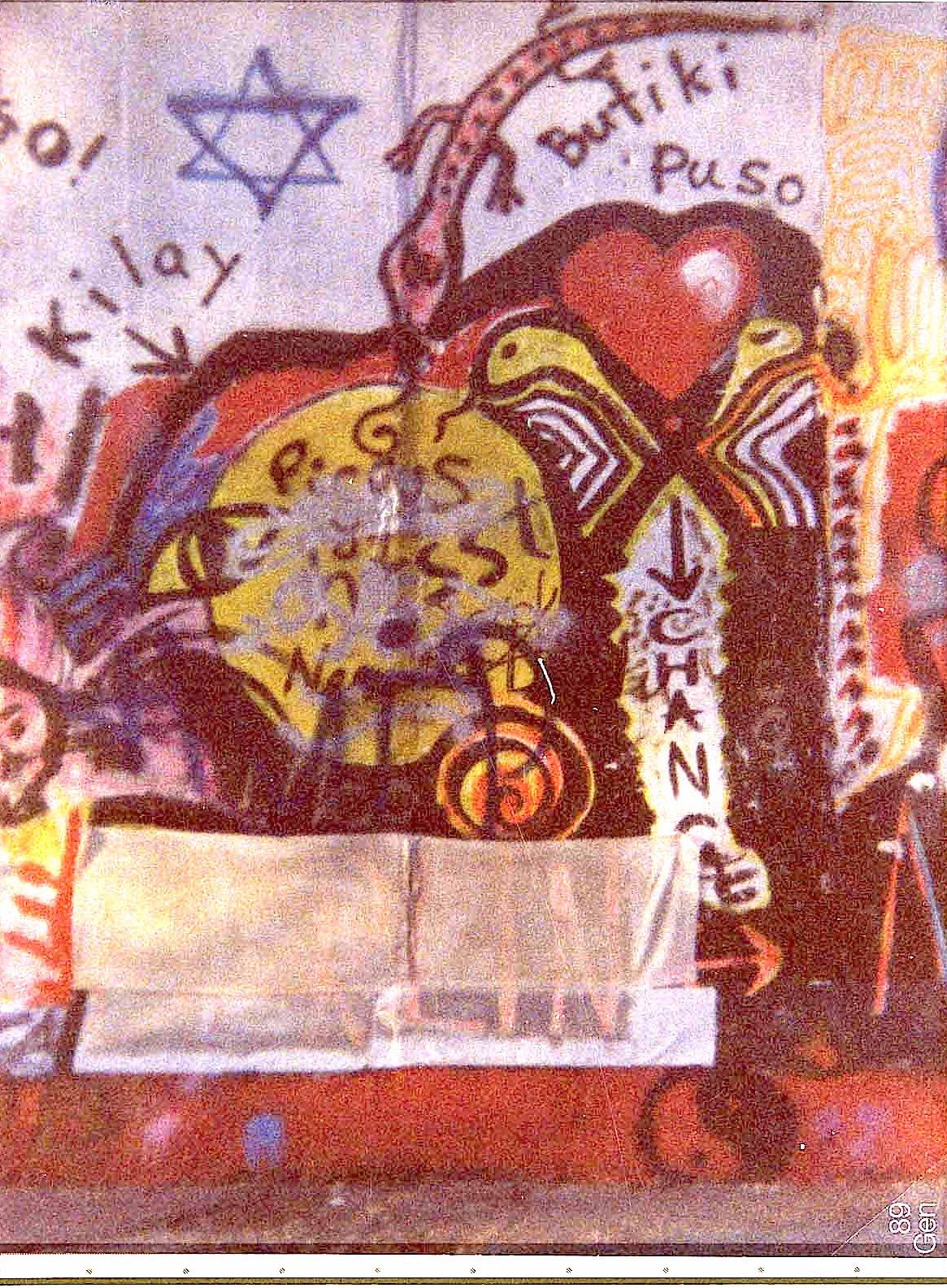This image is a grainy color slide, possibly taken over 25 years ago, showing a heavily graffitied wall. The photograph has a muted palette of red, yellow, blue, light purple, and gray due to its age and lighting conditions. The focal point is a chaotic blend of graffiti layered over what appears to be an original mural. Prominent elements include a large yellow circle with various designs, such as a heart and swirling orange and black patterns surrounding it. There is a red salamander, approximately the length of an arm, curving from the right side into the center of the image. The upper left features a black Star of David. Scattered text includes "Boutique Pousseau," potentially obscured by other tags, with words like "Kile," "change" or "chance," and what might be "Kalay" or "KRLIN." The bottom right corner contains a white "coexist" symbol on a black circle, set against a red background. The overall scene is chaotic and vibrant, with both intricate designs and random graffiti elements merging into a dense tapestry of urban artistry.